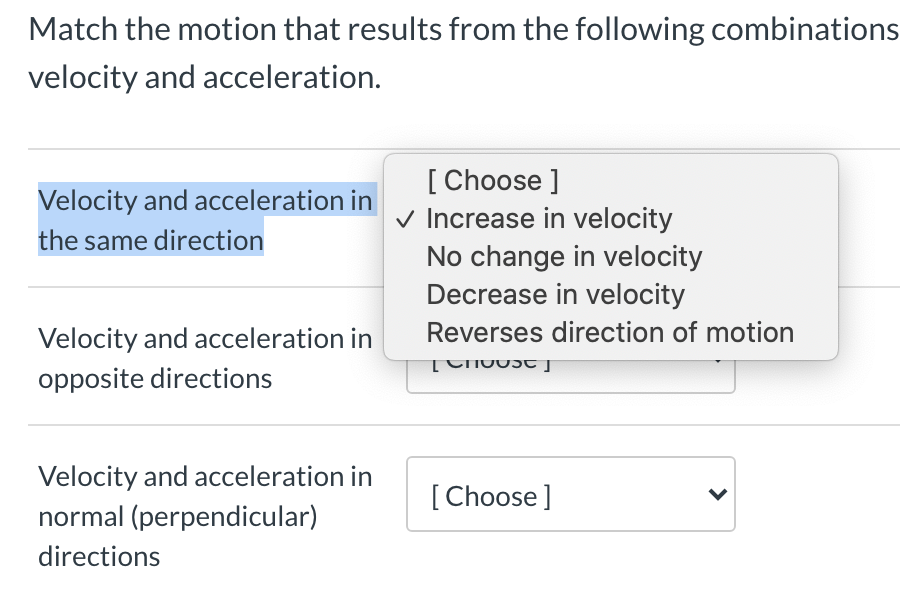**Image Description: Mechanisms of Motion Interface**

The image depicts a user interface related to the study of motion, specifically the outcomes of different combinations of velocity and acceleration. The interface is divided into four distinct sections, each with its own descriptive header and corresponding interaction elements.

1. **Header Section**:
   - The prominent heading reads: "Match the motion that results from the following combinations: Velocity and Acceleration," displayed in a noticeably larger font than the rest of the text.
   - Beneath the heading, a thin gray line separates it from the subsequent content.

2. **Velocity and Acceleration in the Same Direction**:
   - This section is highlighted in a light blue color.
   - It reads: "Velocity and acceleration in the same direction."
   - An overlay box contains a drop-down menu with the following options:
     - Increase in velocity (checked)
     - No change in velocity
     - Decrease in velocity
     - Reverse direction of motion
     
3. **Velocity and Acceleration in Opposite Directions**:
   - Positioned on the left-hand side of the interface.
   - Reads: "Velocity and acceleration in opposite directions."
   - This section also contains a truncated view of another drop-down menu labeled "Choose," partially obscured by the overlay box from the previous section.

4. **Velocity and Acceleration in Normal Perpendicular Directions**:
   - Marked by another thin gray line below the previous content.
   - It states: "Velocity and acceleration in normal (perpendicular) directions."
   - Adjacent to the text is another drop-down menu labeled "Choose."

The overall design suggests an educational tool aiming to demonstrate how different combinations of velocity and acceleration affect motion, with interactive elements for user input to check their understanding of the concepts.